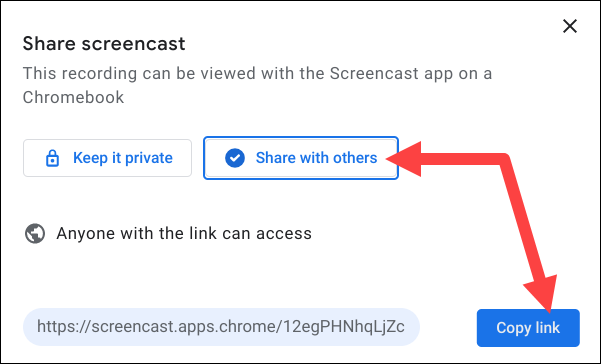The image displays a pop-up dialogue box typical of a screencast sharing interface on a Chromebook. At the top is a black "X" button on the right for closing the pop-up. The main message of the box reads "Share Screenshot" and "Share Screencast," found prominently in a larger font.

Below this, there is a notification stating, "This recording can be viewed with a screencast app on a Chromebook." The dialogue offers two sharing options: "Keep it private," represented by a green lock icon button, and "Share with others," denoted by a blue button with a blue check mark. A red arrow points from "Share with others" down to a "Copy Link" button, indicating a method to share the screencast via a link. The "Copy Link" button is also blue, emphasizing the interactive element.

Additionally, there is an icon of a globe signifying that "Anyone with the link can access" the screencast. Near the bottom of the pop-up, the web address for accessing the screencast is provided as "https://screencast.apps." The arrangement of the elements and the clear visual indicators guide the user on how to share their screencast effectively.